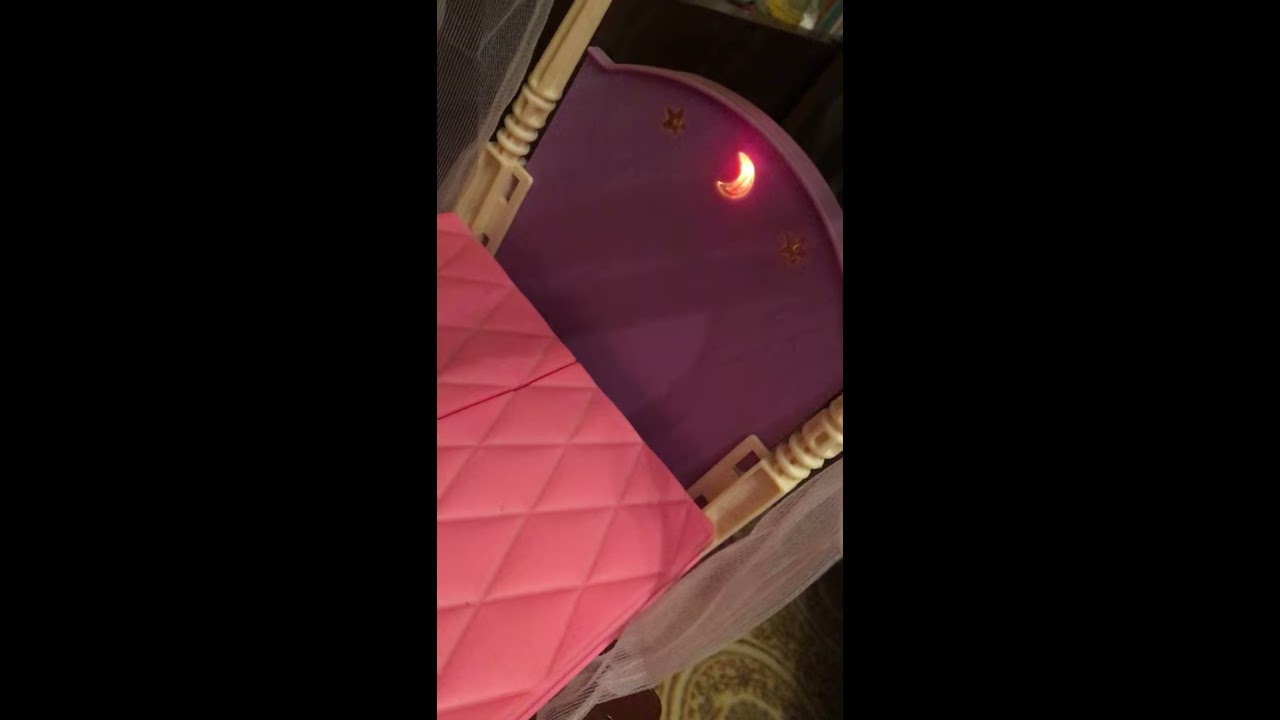This is a photograph of a plastic chair or crib-like object taken indoors in portrait orientation. The object is positioned in the middle of the room, but only a portion of it is visible in the close-up shot. The seat surface is a bubblegum pink color, featuring a line down the middle and diamond-shaped imprints. On either side of the seat, there are cream-colored posts with slots in them, which may be part of the chair's or crib's supportive structure.

The back of the object is purple, resembling a headboard, and it features a decorative theme of stars and a crescent moon. The moon-shaped crescent is located at the top center of the back panel and is lit up with a yellowish or peachy light. On either side of the moon, there are star-shaped cutouts—one to the left and one to the right. The back panel is curved at the top and is supported by white pillars. 

In the background, the floor can be seen, covered with a brown and cream designer carpet or possibly linoleum. Additional details include two vertical black borders on the left and right sides of the photograph, and gauzy fabrics hanging down beside the headboard-like back panel.